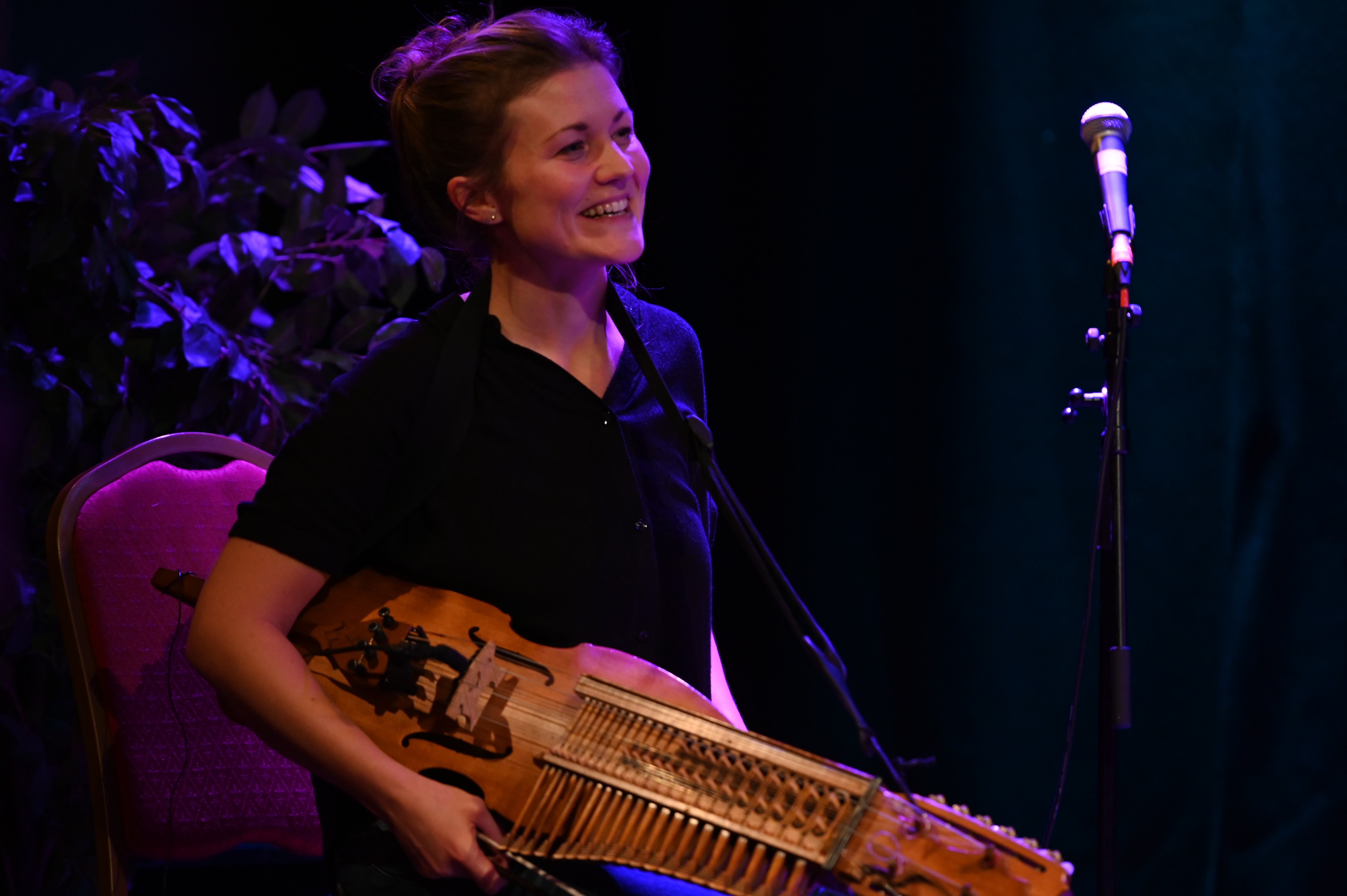The image depicts a white woman standing on a dark stage, smiling gently as if she is performing. She is wearing a black collared shirt and has her hair styled in a short bun. A gray microphone on a black stand is positioned in front of her. The woman holds a unique wooden stringed instrument under her right arm, appearing similar to a viola but larger, with two rows of prongs or sticks covering the strings and a black bar below them. The instrument, which also has a strap over her right shoulder, resembles an intricate mix between a guitar and a violin. She holds a bow in one hand and has a handle over her left shoulder. Behind her, the background is a dark stage punctuated by a pink velvet chair with a metal handle and decorated with plant leaves. There's also a purplish light casting a shiny effect, enhancing the performance atmosphere.